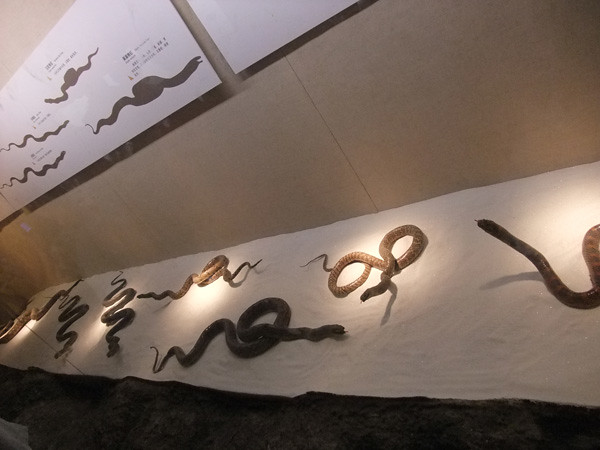In the image, we observe a museum exhibit showcasing various snakes, possibly in a natural history or zoological museum. The backdrop is a cream or brownish-colored wall adorned with detailed posters or diagrams that depict silhouettes of different snake species. Above these illustrations, there is black text providing information about each snake. In the foreground, on a sandy or cloth surface—possibly a table or exhibit panel—there are seven snakes. These snakes are in diverse colors, ranging from brown to black, and some exhibit stripe patterns. The snakes appear lifelike, with some coiled up while others extend their necks upwards or move around. The exhibit is lit by overhead lights casting shadows beneath the snakes, adding to the realistic effect. There is also a large black area at the bottom of the image, which could be part of the background or beneath the exhibit setup, though its purpose is unclear.